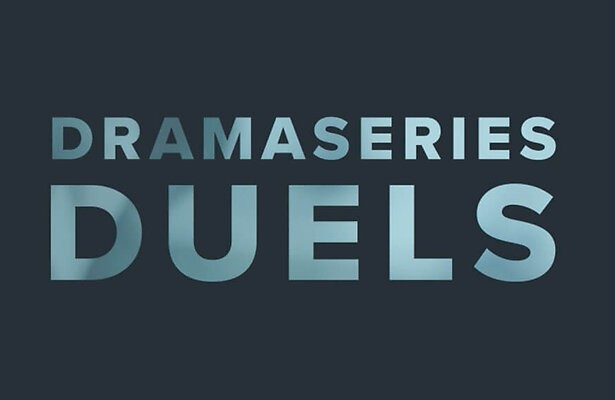The image is a basic banner with a dark blue rectangular background, where the horizontal sides are approximately twice as long as the vertical sides. Dominating the center are two lines of text, each a single word, arranged with "DRAMA SERIES" on the top line and "DUELS" on the bottom line. Both words are written in large, bold, uppercase fonts. "DRAMA SERIES" is in medium-sized letters, while "DUELS" is presented in larger letters. The text is colored in a gradient that transitions from a darker hue at the edges to a lighter blue towards the center, adding a sense of depth and contrast to the words. This gradient effect results in the letters "D" and "A" in "DRAMA SERIES" appearing darker, while the rest of the letters lighten towards the middle before darkening again towards the edges.